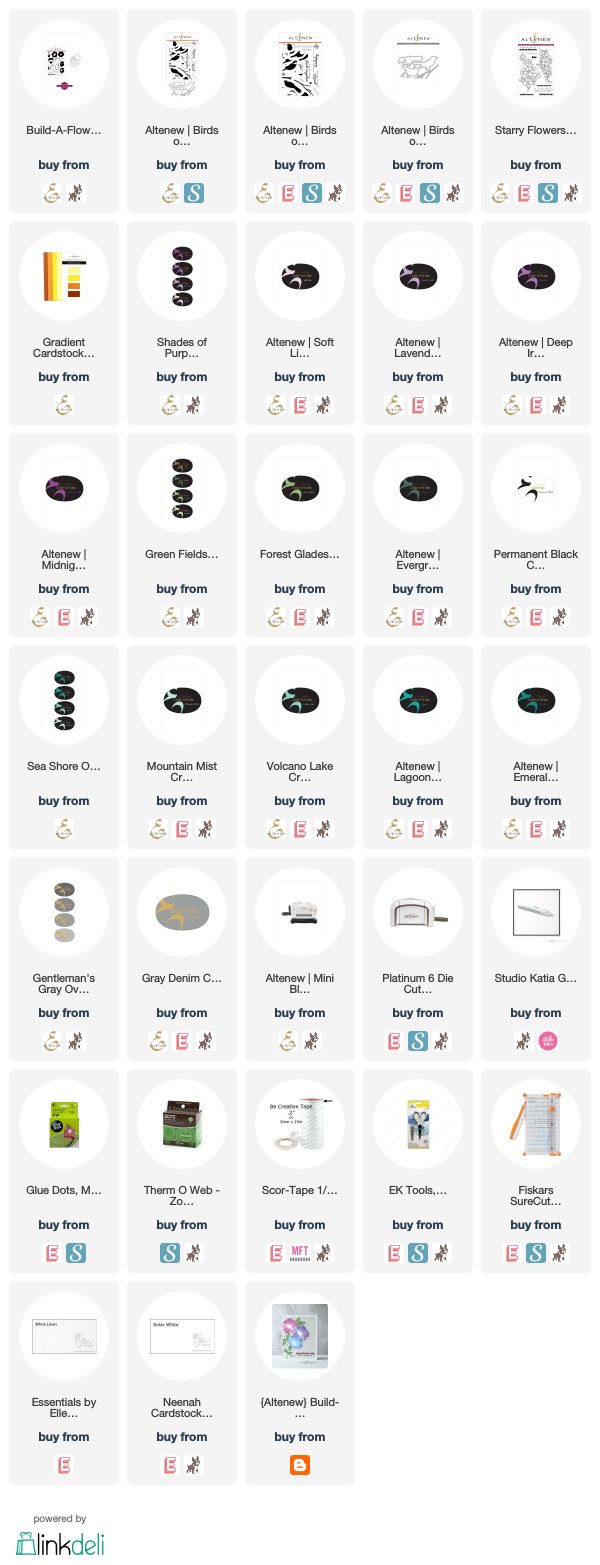This is a cropped screenshot of an online marketplace showcasing 33 products. The layout features 7 rows of items, each presented in small grey boxes. At the top of each box, a white oval frame displays a thumbnail image of the product. Beneath the thumbnail, the product name is clearly labeled, followed by a prominently placed "Buy Now" icon. Directly below this, small icons of various social media apps are lined up. Each of the first 6 rows contains 5 products, while the 7th and final row at the bottom of the page has only 3 items. In the bottom left corner of the page, there is a logo icon for "Linkdel," indicating that the marketplace is hosted or presented by Linkdel.